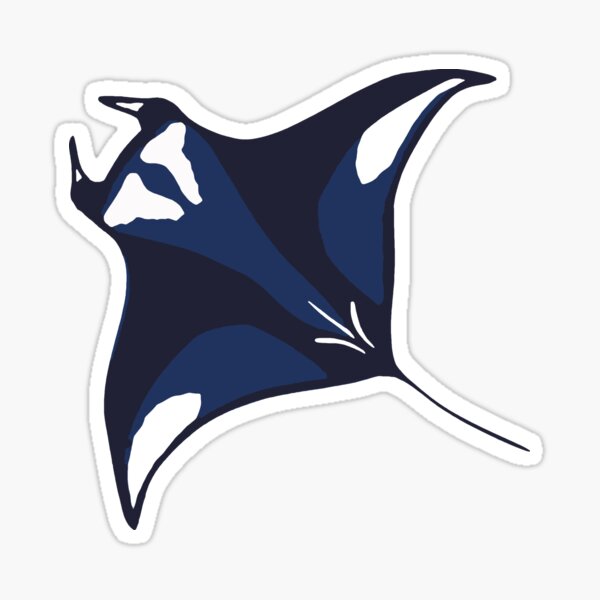In this digital graphic, the central object is an animated stingray, positioned diagonally with its tail pointing toward the lower right and its head angled to the upper left. The background is a neutral gray. The stingray features a blend of dark navy blue, lighter blue, and white, with white accentuating its wings and outlining its form. This image, possibly designed as a sticker or logo, is quite detailed and covers almost the entire frame, showcasing a dynamic and vivid illustration.